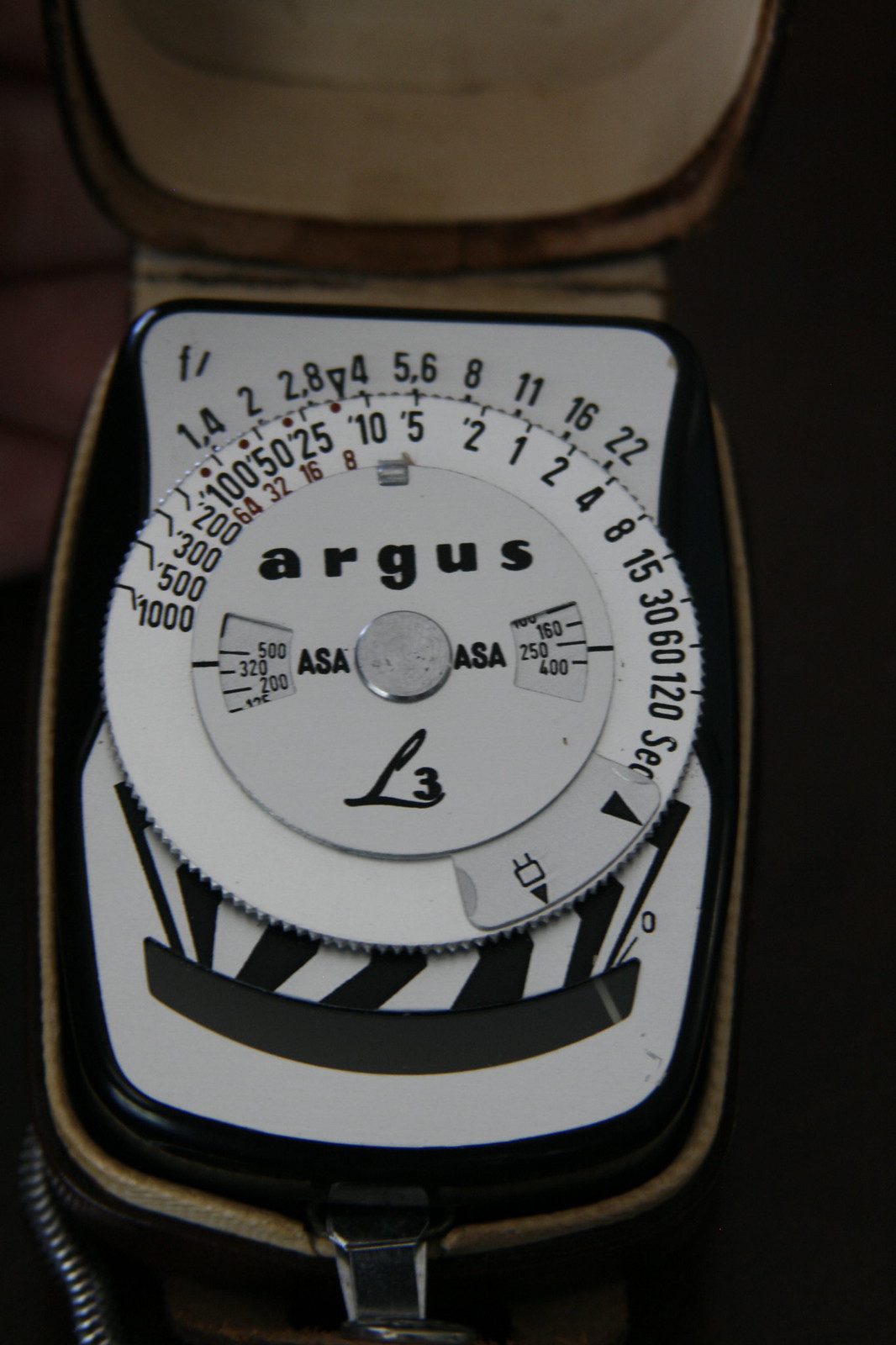This close-up photograph features an Argus light meter, a device crucial for determining correct photographic exposure by measuring light. The light meter, which is predominantly black and white, is rectangular with a central circular dial. This dial is adorned with a series of numbers corresponding to shutter speeds, ranging from 1,000 to 1 second, and even lower values such as 2, 4, 8, 15, 30, 60, and 120 seconds. The top section of the dial lists the f-stop values, from 1.4 to 22, which indicate the aperture sizes. Surrounding the circle are the letters "ASA," representing the film speed. Centrally positioned is the brand logo, displaying "Argus" alongside a distinct "L3" symbol. The meter is housed within a small brown case equipped with a zipper, ensuring its protection.